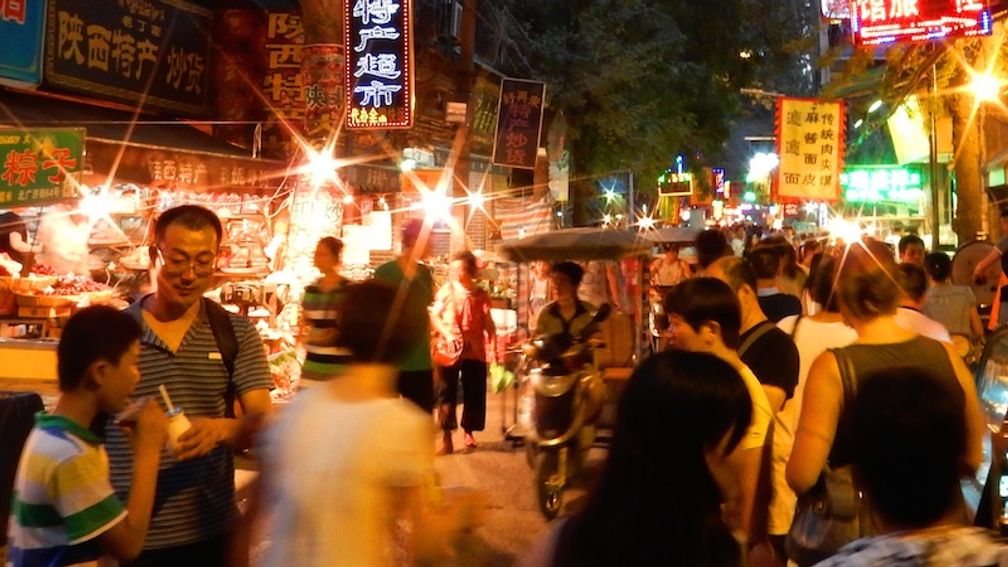The photo vividly captures the bustling atmosphere of a Chinese night market. It is taken at night, filled with bright, colorful lights illuminating the street and vendor stalls. Billboards and signs in Chinese characters, specifically in Cantonese style, adorn the surroundings. Various people populate the scene, some walking, some enjoying food from the market stalls, and others perusing merchandise for sale. In the center of the image, a person rides a motorized scooter, adding movement to the lively setting. A majestic tree with green leaves is visible in the background, adorned with lights that contribute to the vibrant ambiance. The overall energy of the scene is palpable, characterized by the blend of commercial activity, cuisine, and the nightly hustle and bustle unique to street markets in China.